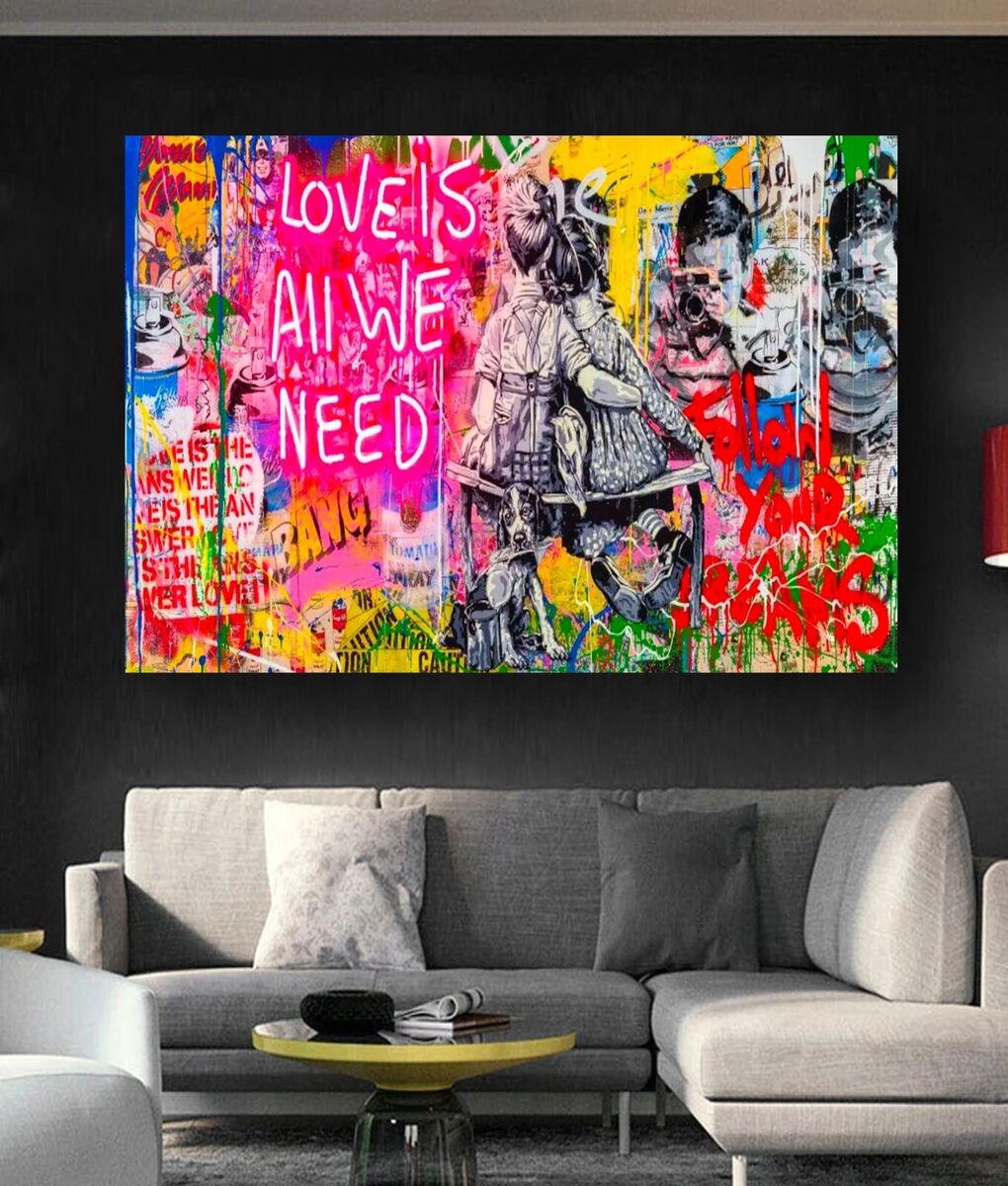This image showcases a modern living room with a contemporary design and vibrant accents. Dominating the room is a substantial, rectangular painting with a graffiti-like aesthetic, hung on a dark-colored wall framed with a light gray upper border. The painting, rich with multiple colors including green, blue, red, pink, white, yellow, orange, gray, and black, prominently features the phrase "Love is all we need" in white, neon-like font against a pink background. This artwork also depicts two children sitting on a bench with a dog beneath them and another child with a camera, seemingly taking a photo. Various graffiti elements such as "bang" and "follow your dreams" add to its eclectic charm.

Beneath the painting, there is an L-shaped, gray fabric corner couch adorned with decorative gray and white pillows, creating a cozy seating area. Adjacent to this couch, on the left, is another white sofa, enhancing the room's luxurious feel. Set against a gray-colored rug is a small, round coffee table with a yellow trim and a glass top, supported by transparent legs. This table, holding magazines, diaries, and black bowls, serves as a central accent in the room. The overall space blends modern comfort with artistic flair, providing both a relaxing and visually stimulating environment.